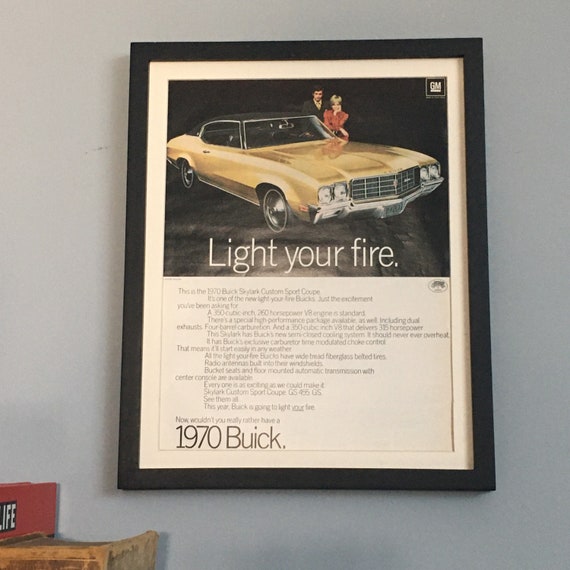The image depicts a framed advertisement from an old-fashioned magazine, likely from the 1970s, showcasing a 1970 Buick. The ad features a gold or yellow Buick, which may have a black convertible roof, with its passenger's side and front visible, and a man in a dapper black suit, along with a woman in a striking low-red outfit, standing on the driver's side. The woman, who has blonde hair, is leaning over the car, positioned where a driver's side mirror would be, with her hand thoughtfully placed on her chin. The background of the top portion of the ad is black, with the letters "GM" prominently displayed in white at the top right. The slogan "Light Your Fire" appears prominently beneath the car, and extensive text below the image details the specifications of the Custom Sport Coupe. At the bottom of the ad, "1970 Buick" is boldly printed in black. The advertisement is hung on a gray wall within a black frame, and in the foreground, a small table holds a red box with the Life magazine logo.